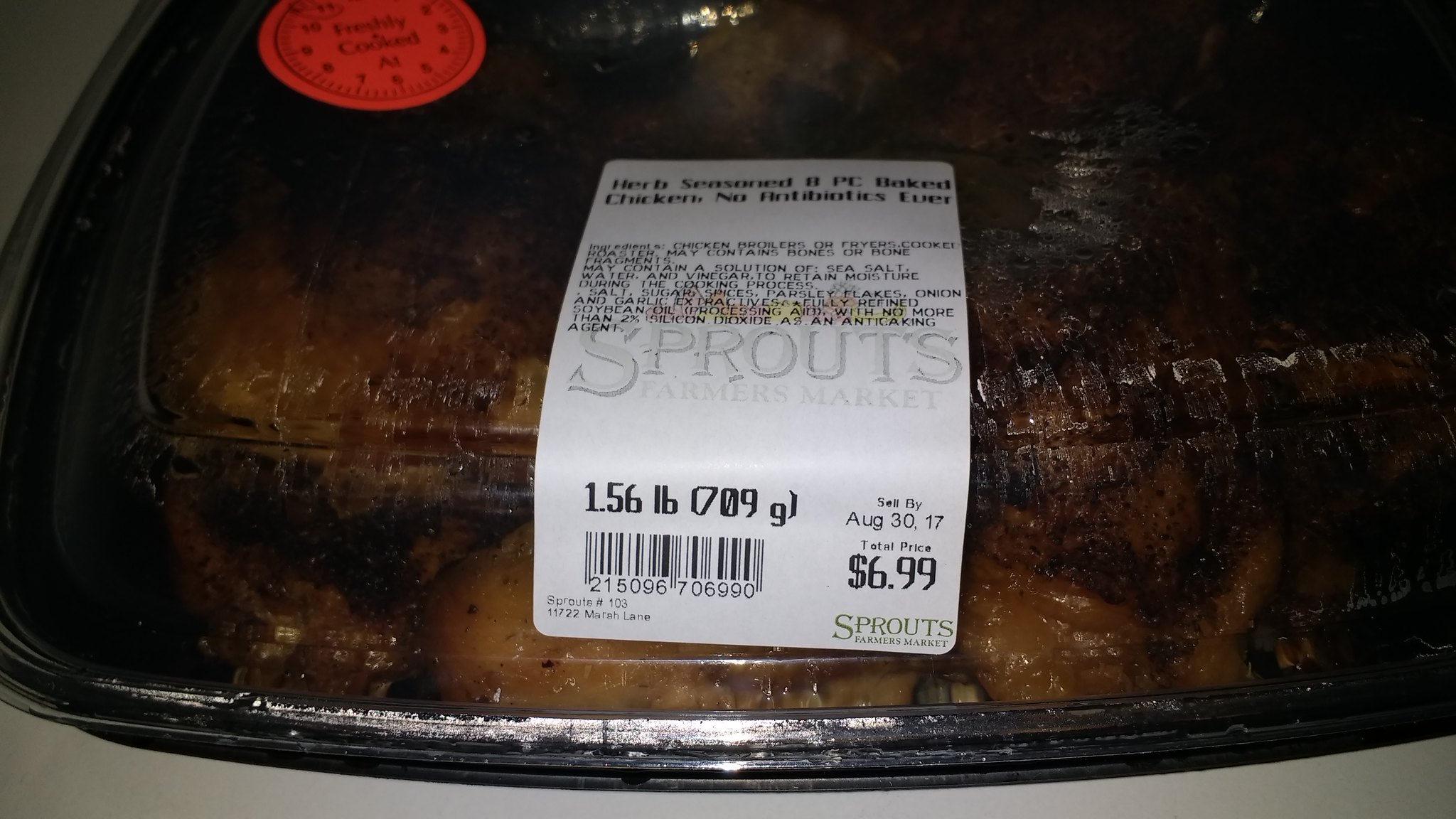In this clear, close-up image, there is a container of herb-seasoned, eight-piece baked chicken from Sprouts Farmers Market. The chicken is packaged in a black-bottom, clear-top to-go box, featuring a prominent white label. The label indicates that the product is antibiotic-free and weighs 1.56 pounds. The sell-by date is August 30th, 2017, and it originates from Sprouts store number 103. The container is placed on a beige-colored counter or shelf, adding a neutral background that highlights the product.